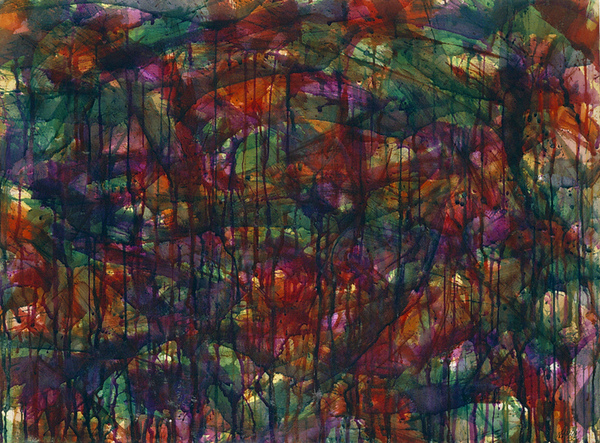The image is a vibrant abstract painting showcasing an intricate interplay of various colors and textures. Dominated by hues of blue, red, purple, and green, the artwork features multiple shades that include hints of gold, orange, and navy, creating a rich and diverse palette. Central to the composition is a series of paint drips flowing from top to bottom, giving the impression of colors cascading down the canvas. These drips form irregular lines and patterns, contributing to a deliberate sense of messiness and fluidity.

In addition to the dripping effect, the painting is interspersed with blobs and blotches of color—red splatters that seem to have been flung onto the canvas, forming spontaneous yet deliberate marks. The colors appear somewhat transparent, reminiscent of glued pieces of tissue paper that allow light to pass through them, yet retain their vividness. Scattered among these colorful elements are crystalline forms that add an extra layer of complexity, blending seamlessly with the other textures.

Overall, the painting abstains from depicting any concrete objects, focusing instead on the aesthetic appeal of contrasting textures and the dynamic movement of the drips and splatters, resulting in a visually compelling abstract composition.